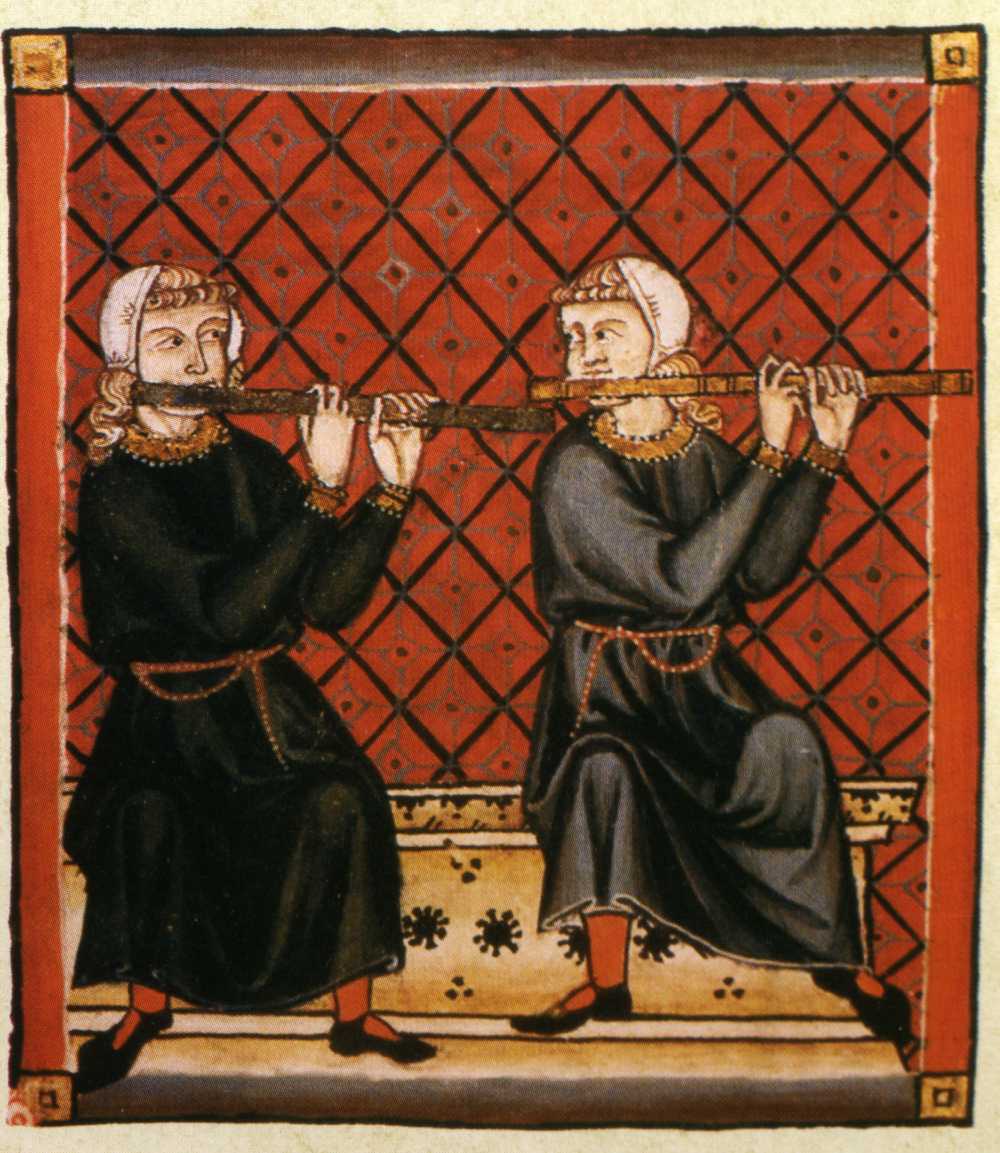The image features a medieval-style ceramic tile with an elaborate, highly detailed scene. Two figures, who appear to be women based on their distinct head coverings and robes, are the focal point. They wear white head coverings that leave their foreheads and hair exposed, accompanied by long black robes with red cuffs and collars, belted with cord-like ribbons around their waists. The women are seated on a low bench or wall and are actively playing long wooden flutes—one darker and the other more golden. Both women have blondish hair, and the one on the left has curly locks. They are dressed in red stockings and black strappy shoes reminiscent of Mary Jane's. The background is dominated by a rich, orangey-red color criss-crossed with black lines forming diamond shapes, each housing intricate patterns. A thin beige border surrounds the image, encased further by a thicker red and black outer border. This detailed, vibrant depiction evokes a strong European, perhaps Dutch or French, medieval atmosphere.